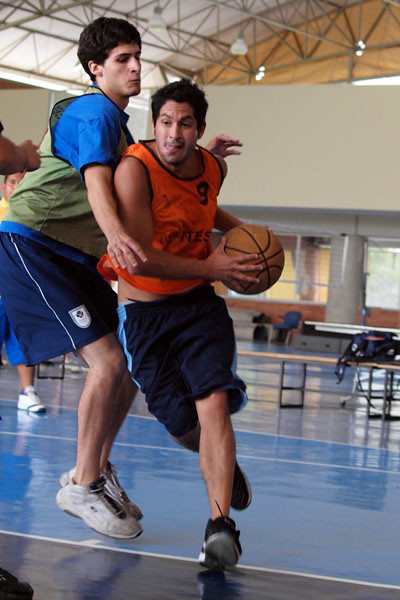In this action-packed vertical portrait taken during a basketball game in a gymnasium, two main players dominate the scene, slightly offset to the left. The central figure is a man in an orange jersey with the number nine, blue shorts, and black basketball shoes. He appears to be Hispanic, with short blonde or brown hair, and is carrying the basketball near his waist, his body slightly turned in an intense action pose, as he rushes towards the basket. Defending him closely is a slightly taller man with short, blackish-brown hair, wearing a blue T-shirt, blue shorts, white gym shoes, and a muted green vest. The gym's blue and gray basketball court gleams under the day-lit rafters adorned with large hanging lights. Surrounding the action, we can observe multiple tables, volleyball nets, benches with bags, and hints of other individuals who appear to be either participating or watching. Despite the fast-paced focus on the two main players, the gym's spacious, structural supports and various elements provide a dynamic and detailed backdrop to this moment of sporting intensity.